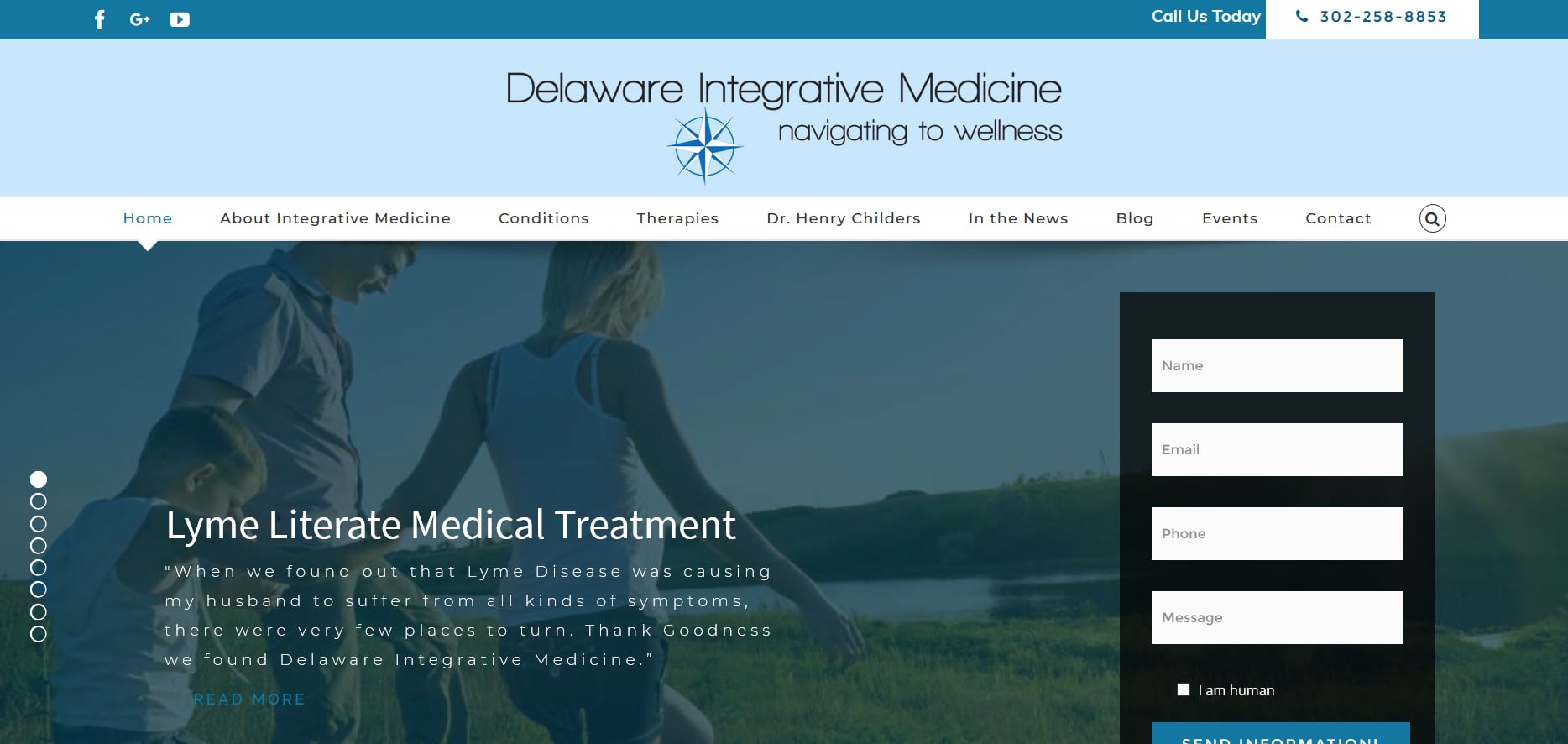The image captures the homepage of the Delaware Integrative Medicine website. At the very top, there is a fine blue border featuring social media icons for Facebook and YouTube, alongside a telephone number positioned on both the left and right sides for easy contact. Below this, a light blue banner showcases the website’s name and logo, accompanied by the slogan "Navigating to Wellness."

Beneath the banner, a navigation menu spans the width of the screen, with headings that include: Home, About Integrative Medicine, Conditions, Therapies, Dr. Henry Childers, In the News, Blog, Events, and Contact. Positioned at the far right of this menu is a search icon for user convenience.

The main section displays an image of a family walking through a field, overlaid with a white text that reads “Limb Literature Medical Treatment." Additional text below this heading provides information about limb disease. This section appears to be part of a series of articles, indicated by eight small dots along the far left side, with the first one highlighted to show the current position in the series.

To the right, a black rectangle presents a form for visitors to enter their name, email, phone number, and message, allowing direct communication with the site’s administrators.